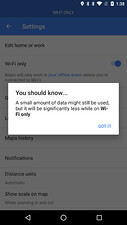A screenshot, taken from a phone, displays the settings menu. In the center of the screen, there is a white dialog box with a message indicating that "a small amount of data might still be used, but it will be significantly less while on Wi-Fi only." At the bottom left of this dialog box, the text "Got it" appears in blue. The surrounding background is dimmed, revealing the notification bar at the top with icons showing Wi-Fi connectivity, approximately half battery life, and a time reading around 1:00. Below the main content, a black navigation bar features three symbols: a left-pointing arrow, a circle, and a square. The darkened settings menu in the background includes options such as "Settings," "Edit," "Home or Work," "Wi-Fi Only," which is enabled, and "Your notifications."